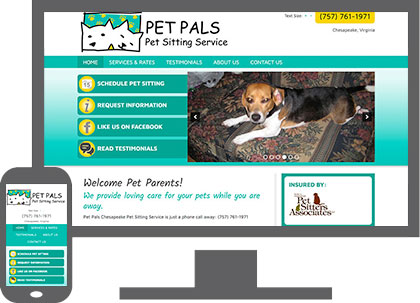The image features a computer monitor displaying the homepage of the Pet Pals Pet Sitting Service website. To the left of the monitor, a smartphone also shows the same website, demonstrating the cross-device compatibility. At the top of the webpage is a whimsical cartoon illustration of a dog and a cat against a vibrant green and yellow background. Beside the illustration, the text reads "Pet Pals Pet Sitting Service."

In the top right corner of the website, contact details are prominently displayed, stating "757-761-1971, Chesapeake, Virginia." Below this, a green menu banner lists navigational options: "Home," "Services and Rates," "Testimonials," "About Us," and "Contact Us." Adjacent to this is a vertical sidebar menu featuring quick links for users: "Schedule Pet Sitting," "Request Information," "Like Us on Facebook," and "Read Testimonials."

To the right side of the screen, a photograph showcases a beagle laying on a floral-patterned rug. The beagle, with its characteristic brown face and white muzzle, white front legs, and a tri-colored body of black, tan, and white, gazes directly into the camera. Below this image, a welcoming message reads: "Welcome Pet Parents. We provide loving care for your pets while you are away. Pet Pals Chesapeake, Pet Sitting Service is just a phone call away, 757-761-1971."

In the bottom right corner of the webpage, a green square outlined in white displays an assurance: "Insured by Pet Sitters Associates."